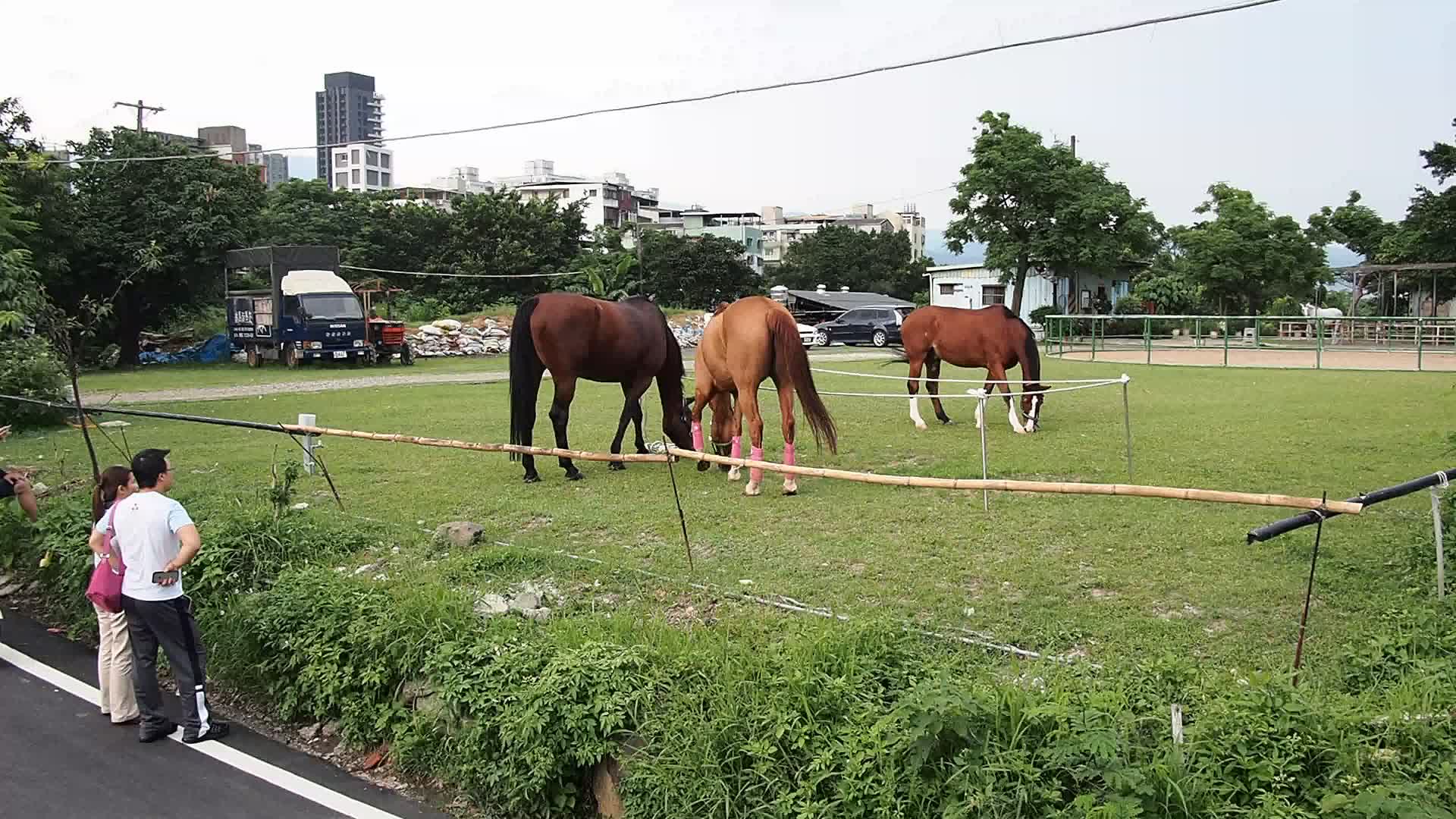In this image, there is a grassy field with three horses of various shades of brown and one white horse in the background. The horses are grazing within a makeshift pen, created by strings tied to metal rods forming a partial enclosure. Observing the horses from the side of a road are two people – a man dressed in a white shirt and black pants, and a woman carrying a pink purse and wearing khakis. In the background, there are several parked vehicles, including an SUV and a truck, suggesting a parking lot area. Beyond the field, the scene extends to city buildings, with a mix of skyscrapers and apartment structures, hinting at an urban setting, possibly in Japan. The sky is overcast, adding a grey tone to the scene, and trees are scattered throughout the background, completing the pastoral yet urban juxtaposition.